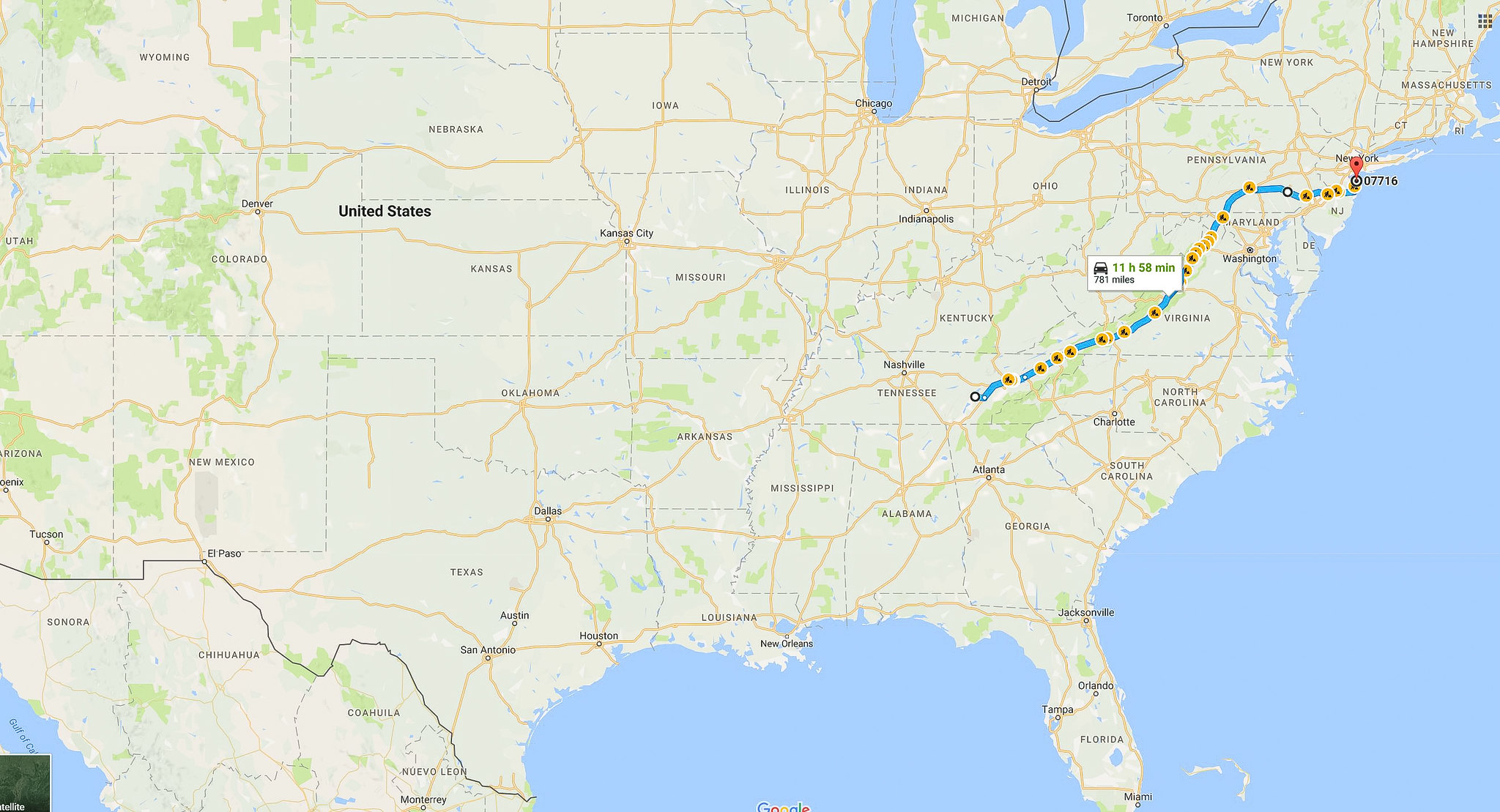This image depicts a detailed map of the United States, excluding the West Coast states like California, Oregon, and Washington. The focus is primarily on the East Coast, Midwest, and southern regions including visible states such as Florida, North Carolina, and Georgia. Prominently featured is a marked route that resembles a traffic or travel map, stretching from New Jersey all the way to Tennessee. This travel line is highlighted in blue with yellow dots, indicating a journey of 11 hours and 58 minutes by car, covering 781 miles. The trail is clearly demarcated, giving the impression of a planned road trip or travel route, and ends at a red pin location. The map’s style is reminiscent of Google Maps, providing clear and detailed visuals of the Eastern and Southern United States.